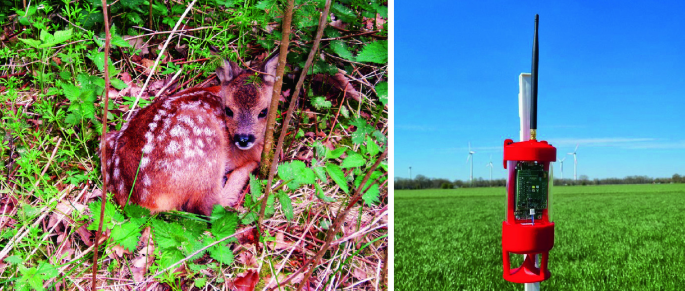The composite image consists of two distinct sections. On the left, there is a rectangular, horizontal shot showcasing a tan-colored baby deer, or fawn, curled up in a resting position. The fawn's back, adorned with white spots, is turned towards the viewer, while its head is looking back over its shoulder. The setting is a woodland area, indicated by the presence of pine straw, dried leaves, and greenery. On the right, the square image features a red cylindrical device with a glass component and a tall, thick black antenna mounted on a white pole. This device is situated in a wide, green grass field with clear blue skies and a few clouds above. The background reveals trees and windmills, suggesting a wind farm environment.